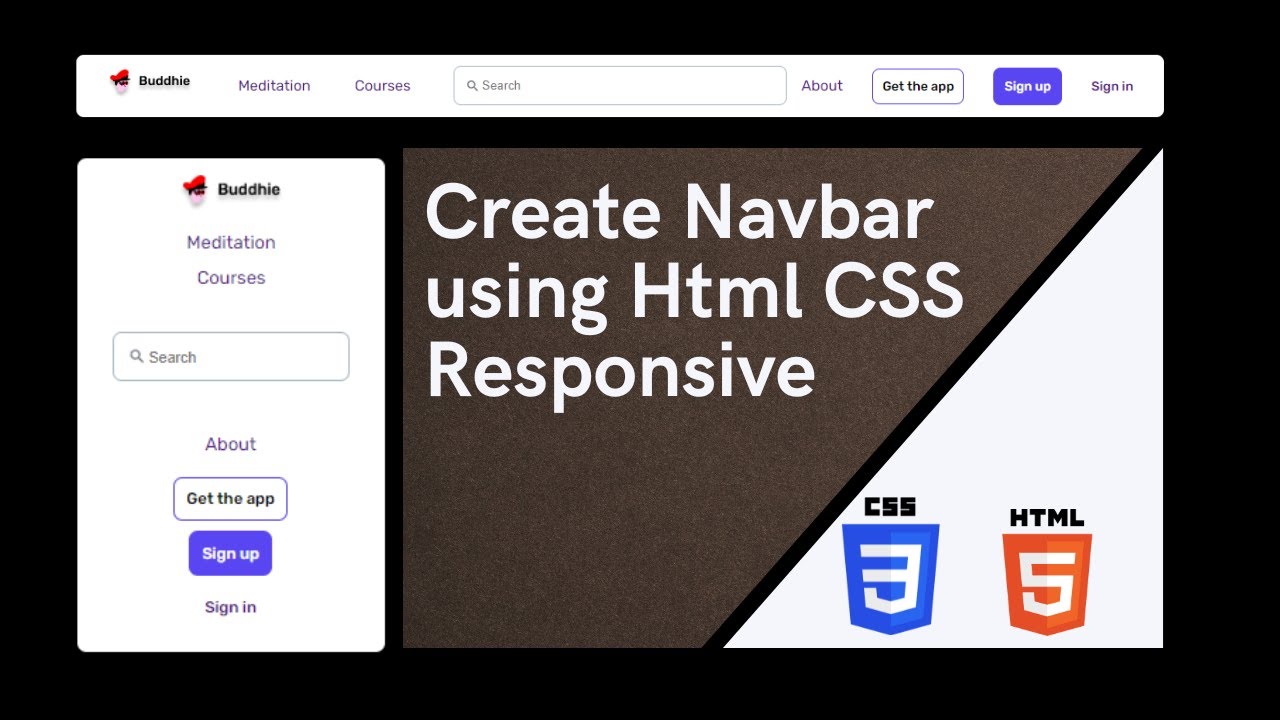The image showcases the homepage of the Budhe website, characterized predominantly by a black background. At the top of the page is a menu bar with a white background, prominently featuring the Budhe website icon. The menu bar offers several options: a search bar with a text entry field, an "About" button, "Get the App," "Sign Up," and "Sign In" buttons.

Below the menu bar, the page is divided into three sections. The left segment, occupying about a quarter of the screen from top to bottom, is dedicated to Budhe Meditation Courses. This section also includes a search bar for text entry, an "About" button, and "Get the App," "Sign Up," and "Sign In" buttons.

The remaining section of the screen, starting just below the top menu bar and extending to the bottom, features a gray background bar divided diagonally into two parts: the top two-thirds and the bottom one-third. The gray area contains white text that reads "Create Nav Bar Using HTML CSS Responsive." In the lower right triangle formed by the diagonal division, there is a white-background box. Within this box, the first area features a symbol with white text on a blue background indicating "CSS." Adjacent to it is an orange symbol with white text indicating "HTML."